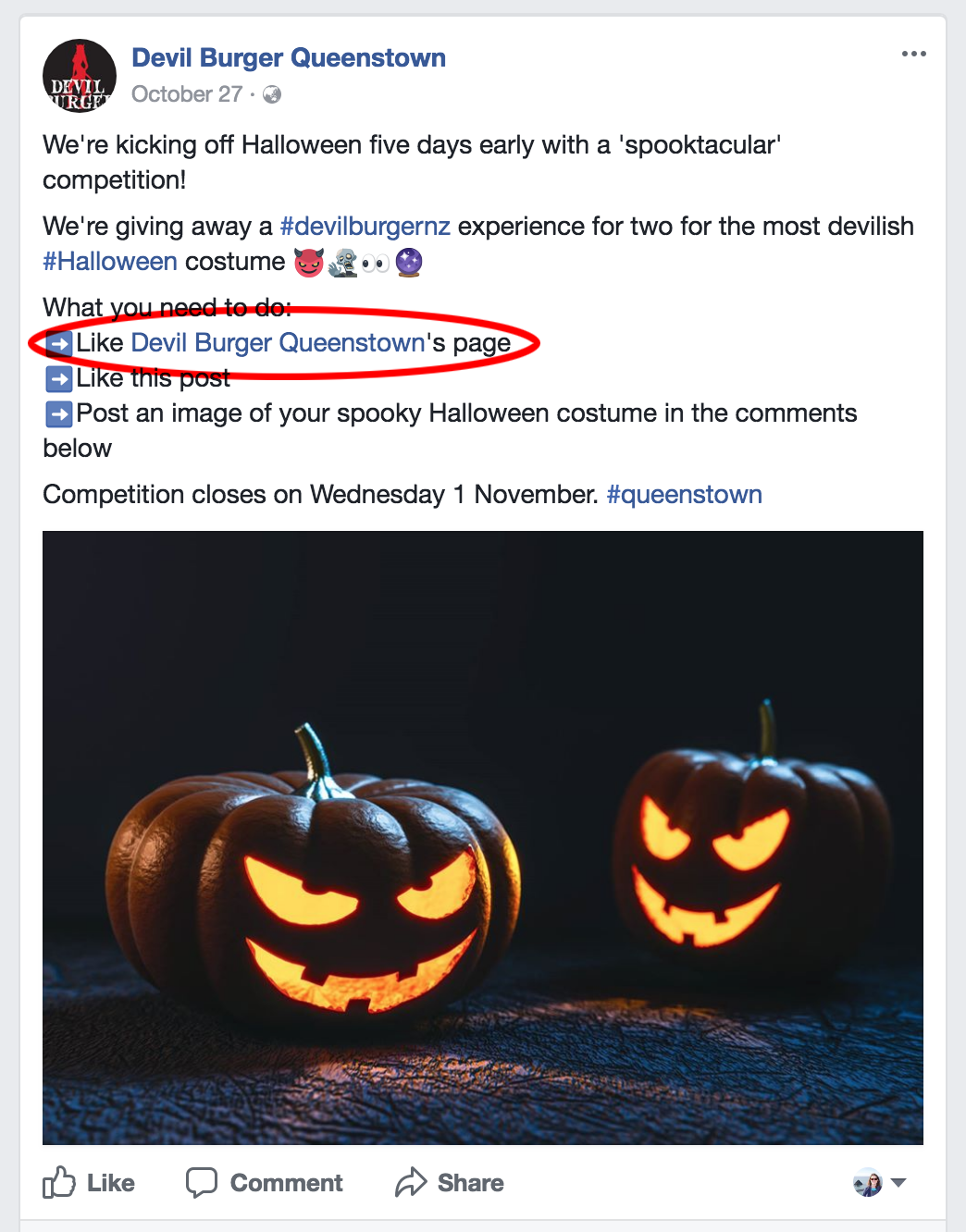Here is a cleaned-up and detailed caption based on the given description:

---

**Caption:** 
Explore our latest social media post from Devil Burger, Queenstown, dated October 27. The post enthusiastically announces their early Halloween celebration with a spooktacular competition, starting five days before Halloween. Participants are encouraged to join by following a few simple steps: 

1. Like Devil Burger, Queenstown’s page (highlighted in red).
2. Like the promotional post.
3. Post a photo of your spooky Halloween costume in the comments below.

The grand prize includes a hashtag Devil Burger and a unique experience for two for the most devilish hashtag Halloween costume. Be sure to enter before the competition closes on Wednesday, November 1. The post features a striking image of two black jack-o'-lanterns with orange illuminated cutouts, creating an eerie yet festive atmosphere.

At the bottom of the post are interactive options for like, comment, and share, each accompanied by respective icons—a thumbs-up for like, a chat bubble for comment, and an arrow for share. Join the fun celebration and show off your Halloween spirit! #Queenstown

**Image Description:** 
A social media post from Devil Burger, Queenstown, prominently features a Halloween competition announcement. The image shows two black jack-o'-lanterns with glowing orange cutouts, enhancing the spooky theme. Instructions for participating in the competition are detailed, encouraging users to engage by liking, commenting, and sharing the post, with icons accompanying each interactive button at the bottom.

---